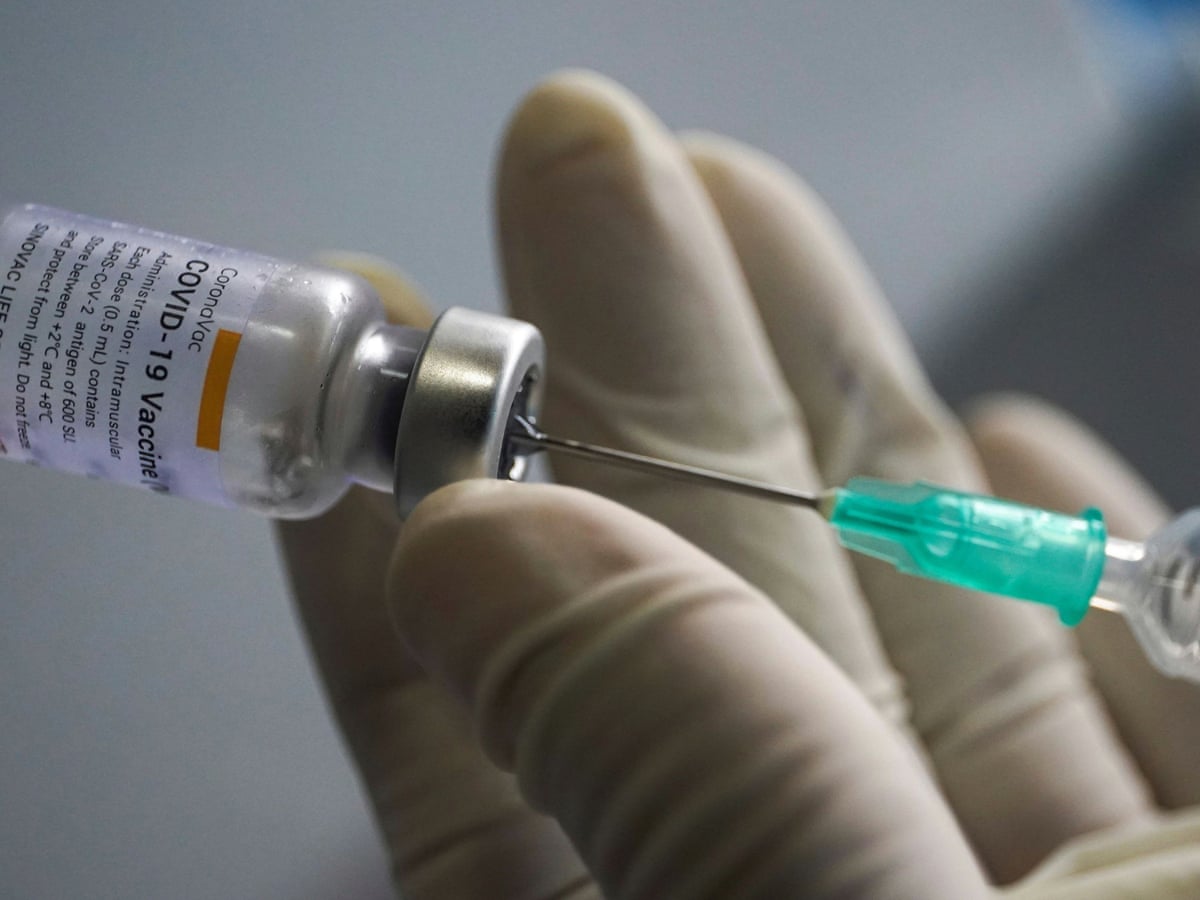In this highly detailed, indoor photographic image, a gloved hand is meticulously preparing a COVID-19 vaccine. The white latex glove partially covering the hand is in the process of filling a syringe from a glass vial. The syringe, featuring a distinctive blue-green hub, is being inserted into the vial's silver metal cap. The vial is labeled "COVID CORONAVAC COVID-19 Vaccine Antigen Track Administration Intramuscular H-Dose 0.5 mL contains SARS-CoV-2 antigen of 600 SIL. Keep between +2° and +8° Celsius, protect from light, do not freeze." The background is blurred, showcasing a neutral gray tone, emphasizing the focal action of the vaccination preparation. This horizontal, rectangular image captures crucial details, emphasizing the precision and care involved in the process of administering the COVID-19 vaccine.